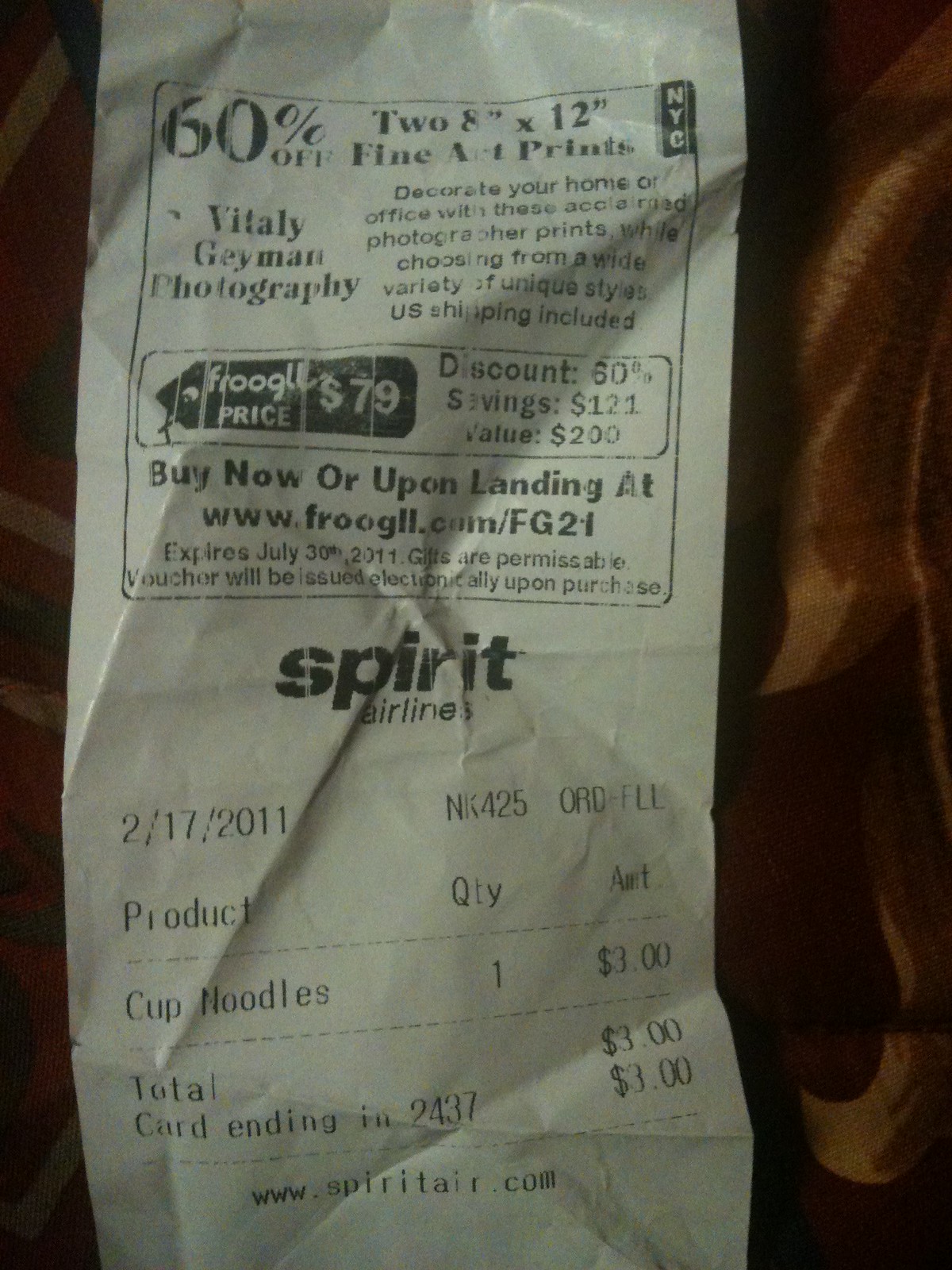The image depicts a crumpled receipt printed on thermal paper, lying on a brown and mottled tan, wrinkled background. The receipt is from Spirit Airlines, dated February 17, 2011. The item listed on the receipt is a single Cup Noodles, purchased for $3.00, bringing the total to $3.00. The amount was charged to a card ending in 2437. At the top of the receipt, there is a 60% off coupon for two 8-inch by 12-inch fine art prints from Vitali Gaiman Photography. The intricate details, from the crumpled texture of the receipt to the mottled background, add depth and character to the image, highlighting both the mundane and the artistic elements of everyday life.